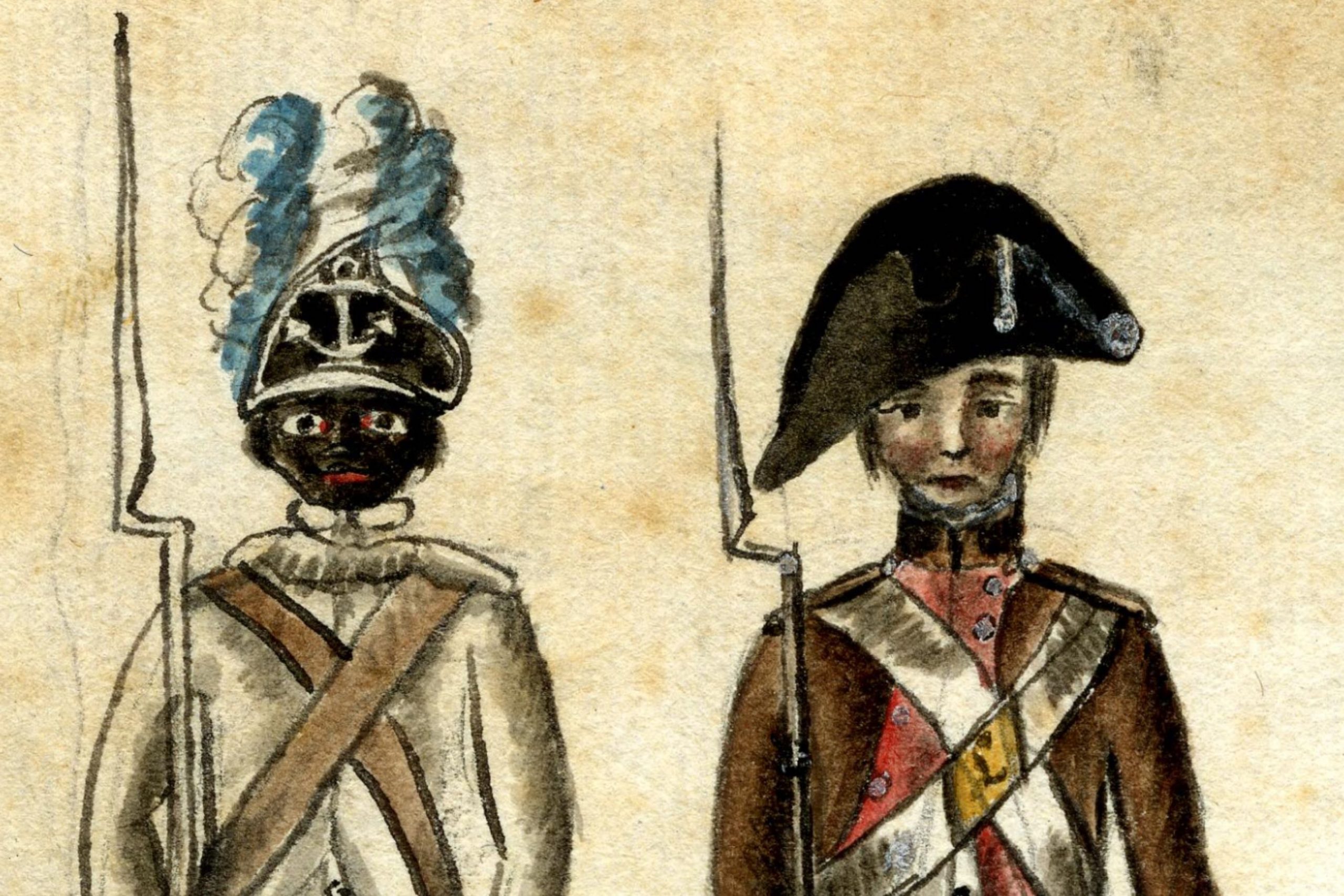The crayon artwork depicts two soldiers standing side by side against a beige background, detailed with uniform elements reminiscent of past centuries. On the left stands a Black soldier in a white uniform, distinguished by a brown cross-strap. His hat, resembling a navy cap, features an anchor and blue and white plumes. This soldier wields a bayonet affixed to a rifle. The right side showcases a White soldier in a brown jacket over a red undershirt, adorned with a white sash that has a golden diamond at its center. His hat is akin to a musketeer’s, tilted and marked with a white line. He too holds a spear-like bayonet. The faces of both soldiers are expressive, with distinctive eyes, lips, and detailed hair or headgear, exemplifying a combination of historical and imaginative military attire.